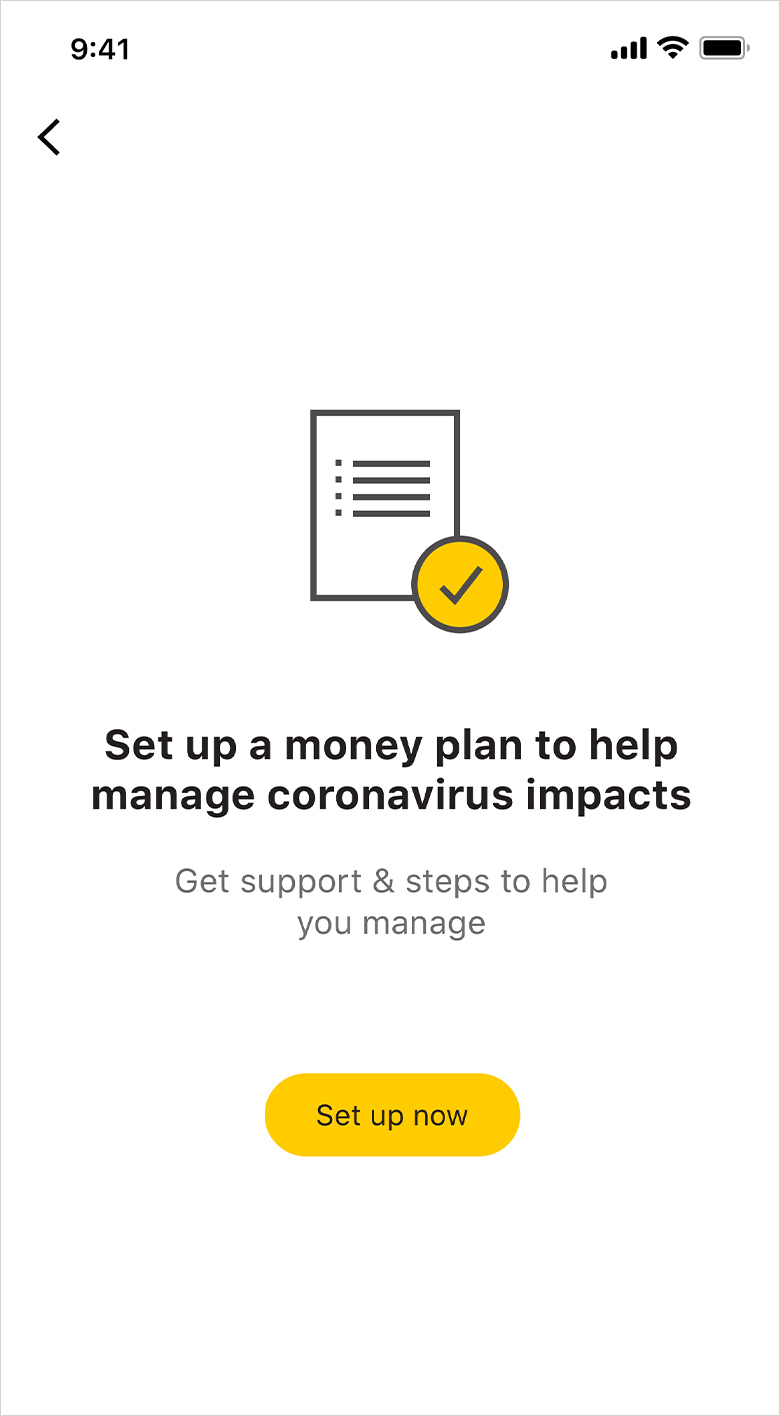This is a detailed screenshot from a mobile phone with a pure white background. The time is displayed in the upper left corner in black font as "9:41". In the upper right corner, black icons indicate the phone's Wi-Fi connection, mobile signal strength, and battery status. Just below the time is a small black arrow pointing to the left.

Dominating the center of the screen is a black icon representing a piece of paper with a bullet list. In the lower left corner of this icon, there is a yellow-filled circle with a black checkmark inside.

Directly beneath the central icon, a bold black font reads: "Set up a money plan to help manage coronavirus impacts." Below this, in gray font, it says: "Get support and steps to help you manage."

Further down the screen, there is an orange oval-shaped button with the text in black font that reads "Set up now," with spaces separating the words.

The entire screenshot is neatly bordered with thin black lines, giving it a clean and organized appearance.